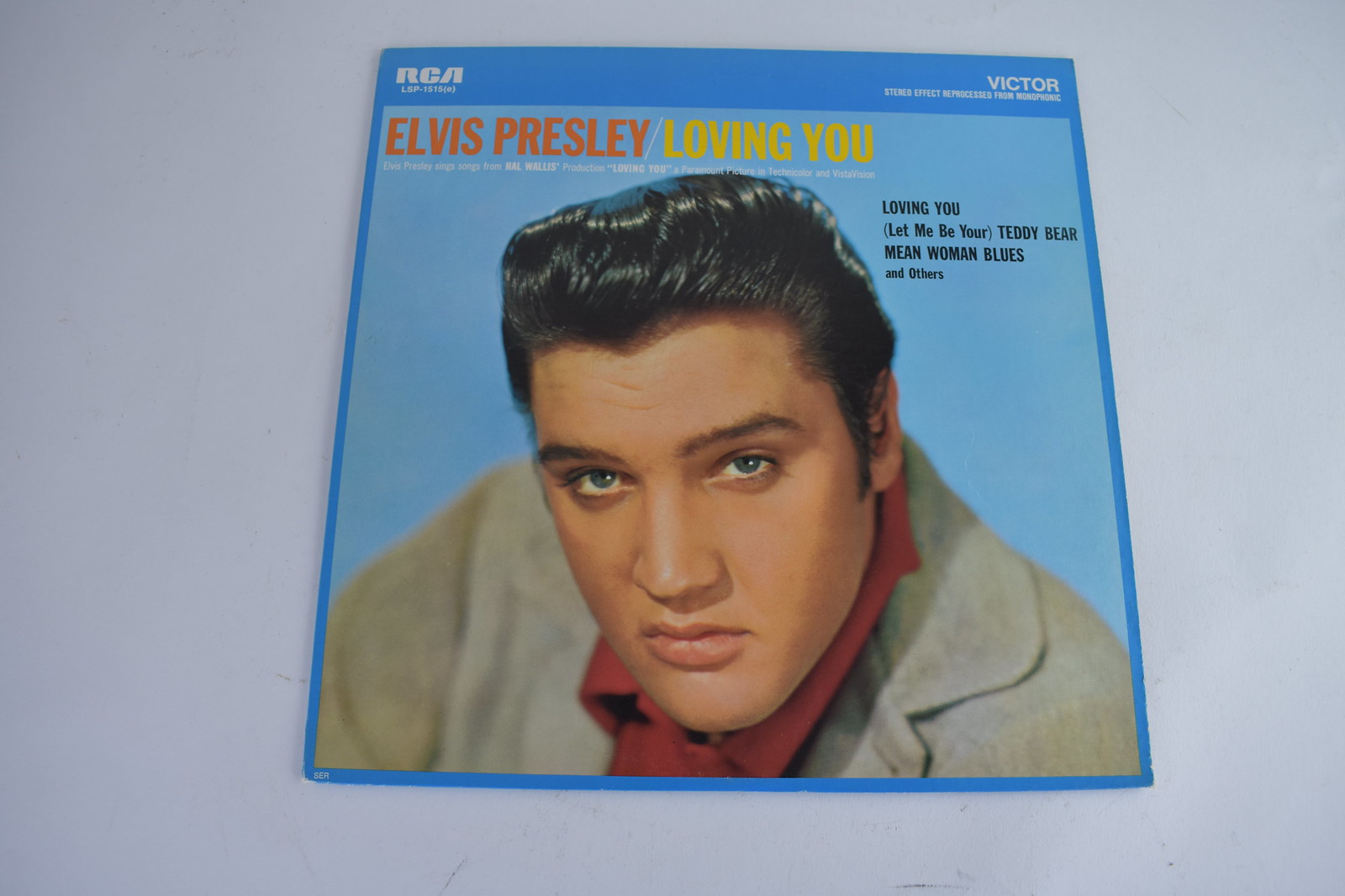This image showcases the album cover for the Elvis Presley single "Loving You," produced by RCA Victor. The cover has a striking dark blue border with a light blue background. A chest-up photo of Elvis Presley dominates the center, where he is seen sneering at the camera with his slicked-back black hair and piercing eyes. Elvis is clad in what appears to be a wool coat and has a red shirt or bandana around his neck. The top banner features both dark blue and regular blue, where "RCA" is in white font on the left and "Victor" on the right. Above Elvis’s face, his name is emblazoned in bold orange font, with the title "Loving You" in yellow font directly below it. To the right of Elvis's head, additional song titles are listed in black font, including "Mean Woman Blues" and "Let Me Be Your Teddy Bear."